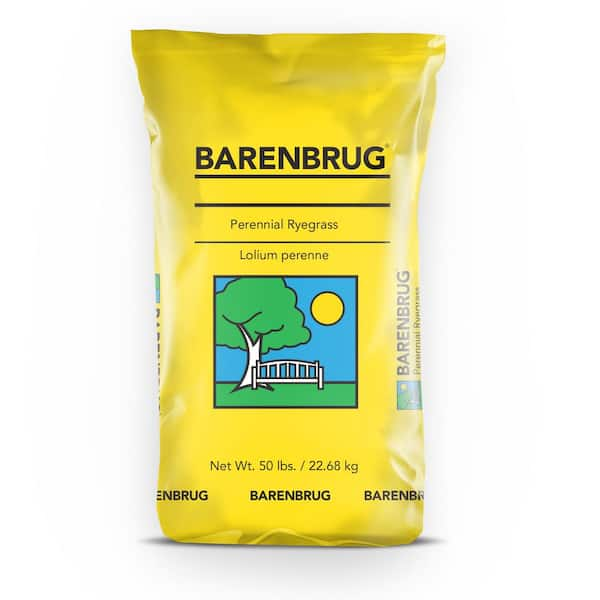A photograph of a yellow bag commonly used for packaging materials like potting soil or grass seed. At the top of the bag, "Barenbrug" is prominently displayed in black lettering above a black line. Below this line, the words "perennial ryegrass" appear, followed by the Latin name "Lolium perenne," also in black. In the center of the bag, there is a cartoon-like square image outlined in black. This illustration depicts a green tree with a white trunk on the left, a gray bench seated on green grass in front of the tree, a blue sky background, and a yellow circular sun in the top right corner. Near the bottom of the bag, the text indicates the net weight as "50 pounds" and "22.68 kilograms." The manufacturer's name, "Barenbrug," is repeated three times across the front of the bag and is also featured on both sides with a partial view of the same park scene.